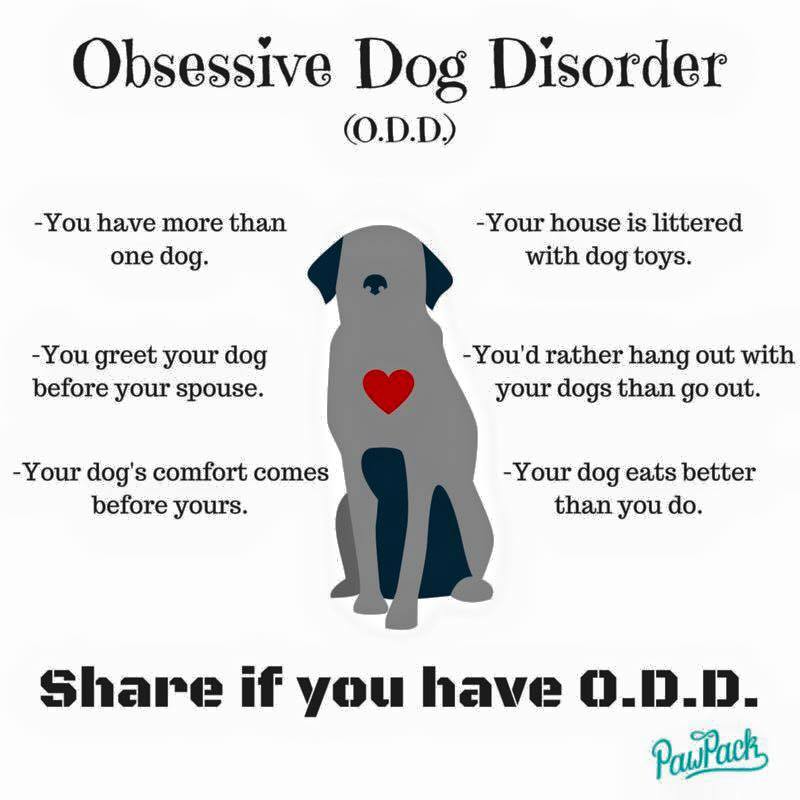The image is a comical depiction of "Obsessive Dog Disorder" (ODD), with a light blue background. At the top, the bold black text reads "Obsessive Dog Disorder, ODD," with the I's dotted with hearts. Below this, there's a stylized gray and blue outline of a sitting dog, featuring a red heart on its chest. The dog has ears and a black snout, with a lighter gray body and a darker gray tummy, but lacks facial features. To the left of the dog are three bullet points: "You have more than one dog," "You greet your dog before your spouse," and "Your dog's comfort comes before yours." To the right, three more bullet points list: "Your house is littered with dog toys," "You'd rather hang out with your dog than go out," and "Your dog eats better than you do." At the bottom, it prompts readers to "Share if you have ODD," followed by the name "PAWPAC" in blue-green text.